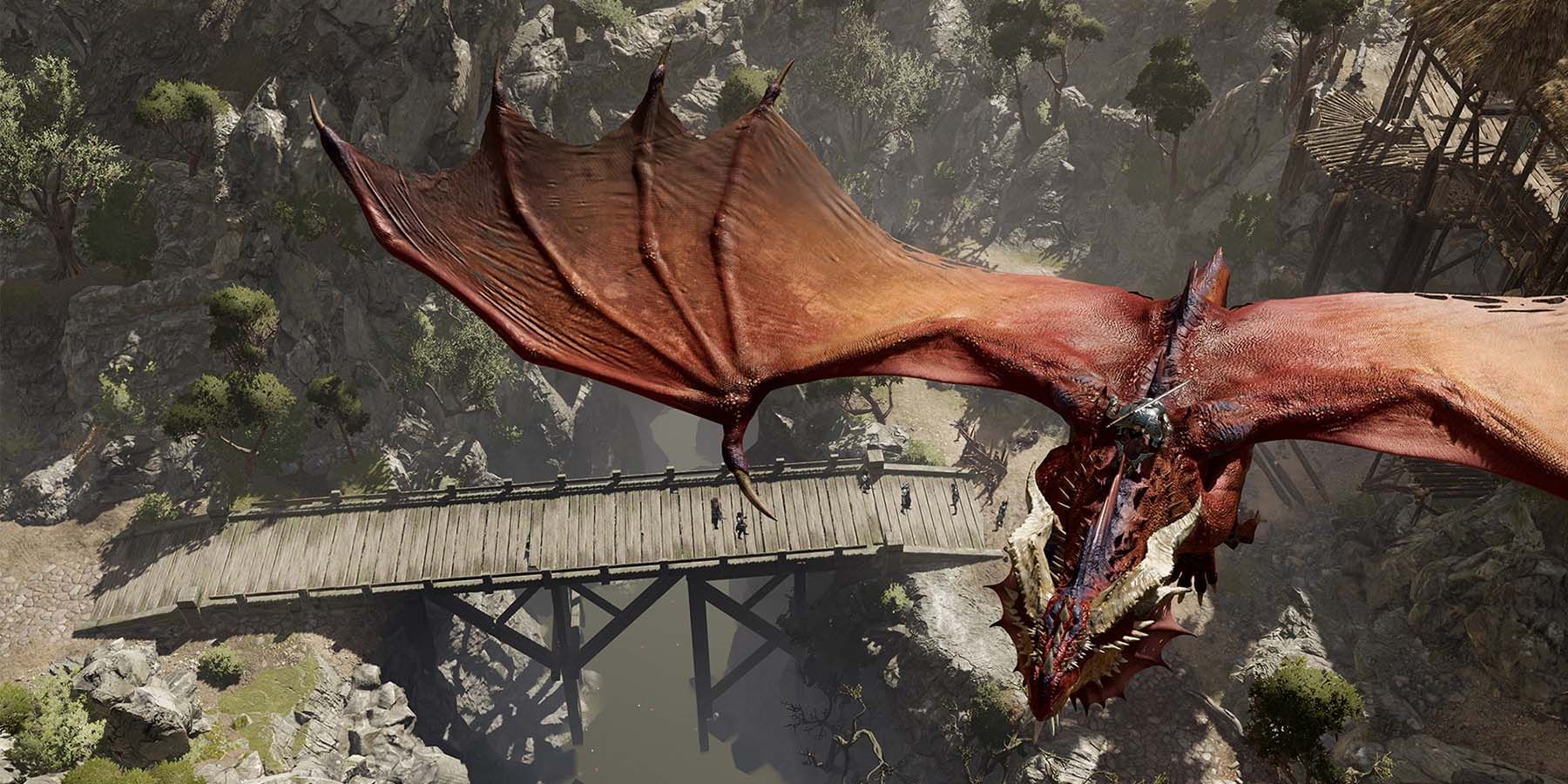This screenshot from an unidentified game offers an aerial view of a dramatic scene centered on a majestic wooden bridge spanning a river nestled between cliff faces. Five people are visible on the bridge, seemingly engaged in conversation or crossing. The terrain on the left side of the image features open land dotted with tall, green trees and scattered rocks, including notable boulders. On the right side, the landscape is dominated by a massive, intricately designed structure that resembles a pterodactyl with brownish wings and a menacing visage. This impressive, potentially AI-generated entity flies above, emitting an eerie presence with its claws emerging from its wings, a round metal object with an ominous needle-like projection on its underside, and horns decorating its head. Below the bridge, the river can be seen with standing water, adding depth to the scene that combines natural beauty with mythical, possibly post-apocalyptic, elements.